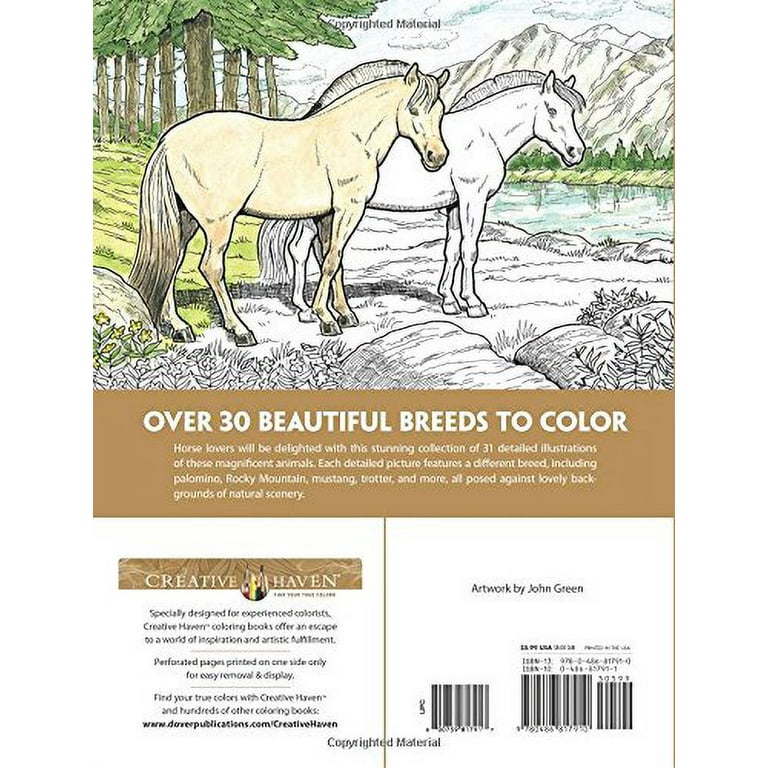This is an image of the back cover of a coloring book. The top half features an illustration of two horses standing on a grassy plain next to a creek, with mountains and trees in the background. One horse is colored light brown, while the other and several elements like mountains and the sky remain black and white. Part of the trees and grass have been colored, with the tree bark in brown and the foliage in green. Above the horses, there is a copyright notice.

Beneath the illustration is a brown rectangular section with the text "OVER 30 BEAUTIFUL BREEDS TO COLOR" in white, uppercase letters. Below this, there's smaller white text that reads: "Horse lovers will be delighted with this stunning collection of 31 detailed illustrations of these magnificent animals. Each detailed picture features a different breed including Palomino, Rocky Mountain, Mustang, Botter, and more. All posed against lovely backgrounds of natural scenery."

In the lower left corner, a rectangular section says "Creative Haven" in white, with some smaller black text underneath it. In the lower right, it says, "Artwork by John Green," with a barcode and UPC code below.